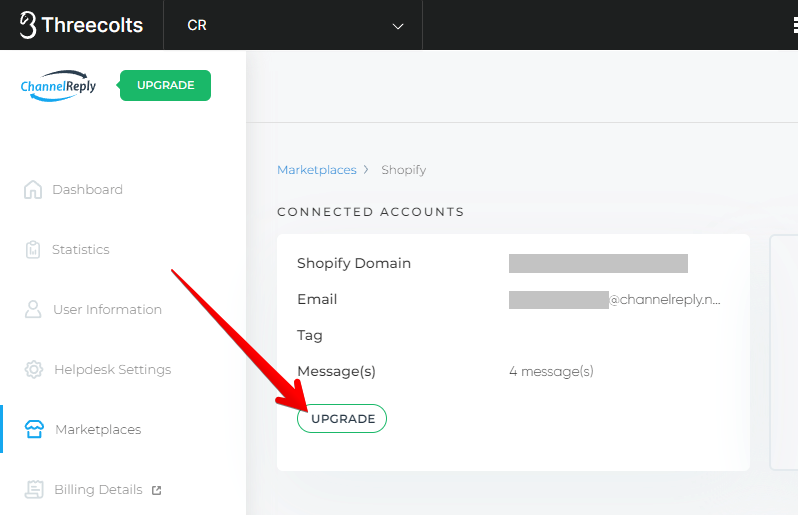The image depicts a webpage from a service or platform named "3 Colts." Positioned at the top left of the black header, the text "3 Colts" is displayed prominently, suggesting it is the title or name of the webpage. Adjacent to this is a dropdown menu labeled "CR." Beneath the header lies a logo for "Channel Reply," accompanied by a prominent green button labeled "Upgrade."

Below the logo and the green upgrade button, there is a navigation menu with several options: Dashboard, Statistics, User Information, Help Desk Settings, Marketplaces, and Billing Details. 

To the right side of the main content area, there are additional navigational elements. At the top, "Marketplaces" is listed, followed by an arrow pointing to "Shopify," indicating a sub-section. Below this, another section titled "Connected Accounts" appears. Further down, headings such as Shopify, Domain, Email, and Tag are visible.

Within this section, there is a line indicating "Messages," showing that there are four messages. A prominently outlined green button labeled "Upgrade" is situated here, with a large red arrow pointing towards it, drawing attention to the option to upgrade.